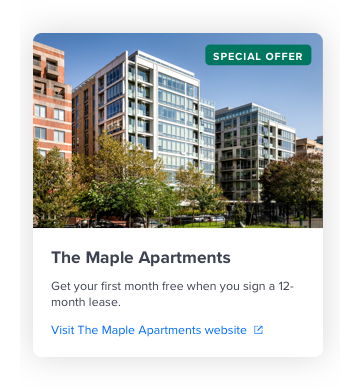This image captures a contemporary cityscape featuring a row of stylish apartment buildings. Prominently displayed are two modern white buildings flanked by two striking red structures. The white buildings appear to be the focal points, boasting sleek, expansive glass facades on one or two sides, allowing for large, pristine windows that suggest a recent construction. Lush trees are planted in front of the white buildings, adding a touch of greenery and possibly indicating a park-like setting, perhaps named Park Lake. A road runs in front of the buildings, completing the urban scene.

Below the buildings, a white banner announces, "The Maple Apartments," followed by an enticing offer: "Get your first month free when you sign a 12-month lease." The message directs viewers to visit the Maple Apartments website, with the clickable link highlighted in blue. A blue box features a pin icon, possibly indicating a location marker.

The background reveals a cloudless, vibrant blue sky, with sunlight softly reflecting off the building surfaces. The surrounding city block stretches out with additional buildings of varying colors but similar heights, creating a cohesive yet varied architectural landscape.